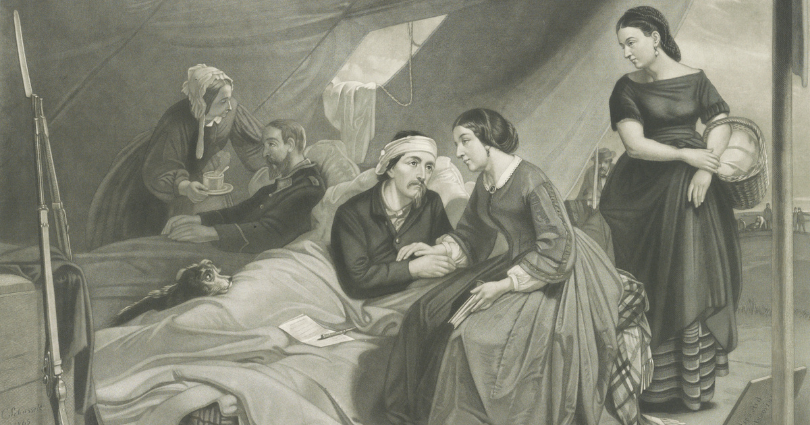The black-and-white painting, designed to resemble an old photograph, portrays a poignant scene inside an army tent, likely from the Civil War era. The artwork is landscape-oriented and vividly details a makeshift military hospital. 

Central to the scene are two men lying in adjacent beds. The man on the right has a bandage around his head, and he looks off to the side while a woman, possibly his wife, sits beside him, tenderly holding his hand. Amidst his belongings are a pen and a piece of paper resting on his bed. A dog lies on his legs, adding an intimate touch to the setting. 

To the left is another bedridden man. A woman, dressed like a maid with a traditional hat, leans over him, offering a steaming cup of tea or coffee. Nearby, military rifles with bayonets are propped against a crate, reinforcing the wartime atmosphere. 

In the background, the opened tent flaps reveal silhouettes of people and tents extending into the distance. Another woman, carrying a basket of cloth, gazes over the scene, contributing to the bustling yet somber ambiance of this historical medical camp.